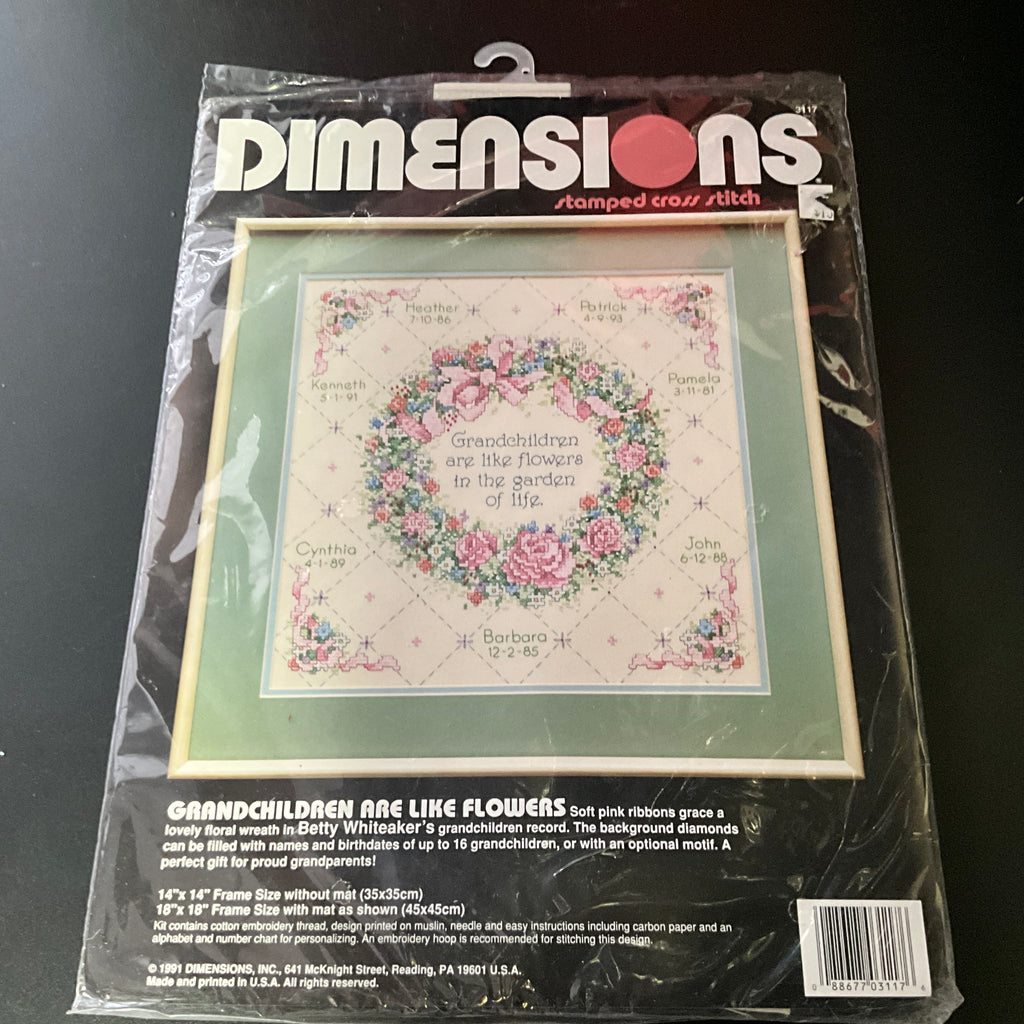This image is a square, color photograph of a Dimensions Stamped Cross Stitch kit. Encased in a plastic bag with a hook at the top, suggesting it is meant for store display, the bag features prominent branding with the company name, "Dimensions," where the "O" is depicted as a red circle. Below the brand name, the product type ("Stamped Cross Stitch") is written in red, and further text in white reads, “grandchildren are like flowers.” The kit is designed as a gift for proud grandparents and showcases a flowery motif with soft pink ribbons gracing a lovely floral wreath. 

The central design includes diamonds that can be personalized with the names and birthdates of up to 16 grandchildren, or an optional motif, and features text that reads, "grandchildren are like flowers in the garden of life." The displayed sample names include Petrie, Pamela, John, Barbara, Cynthia, Kenneth, and Ed alongside their birthdates. 

At the bottom, it details the contents of the kit: embroidery thread, a design printed on muslin, a needle, easy instructions, carbon paper, and an alphabetical and number chart for personalizing. It notes that the design fits a 14 x 14-inch frame without a mat or an 18 x 18-inch frame with a mat. The photograph also includes a barcode on the lower right corner and additional manufacturer information, including the address and that the product is made and printed in the USA. The entire design is framed with light brown wood and features additional floral elements and ribbons at each corner.